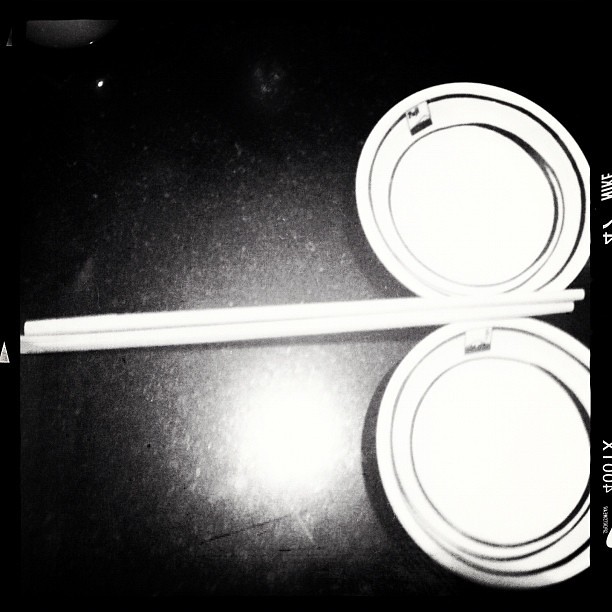This is a black and white photograph taken in a dark setting with a camera flash effect that illuminates the scene, giving it an artistic and almost abstract quality. The background appears to be a black, marble-like surface, and the light in the middle of the frame gives it a dynamic look. In between two bowls that sit on the right-hand side of the image, there are two long, thin sticks that resemble chopsticks or possibly drumsticks running horizontally across the photo. The bowls themselves are light-colored with dark, concentric circles and a black swirl pattern connecting them. A partially visible black border around the photo includes some white lettering and numbers, likely indicating the model of the camera used, which appears to be a Nike 4T0TX.